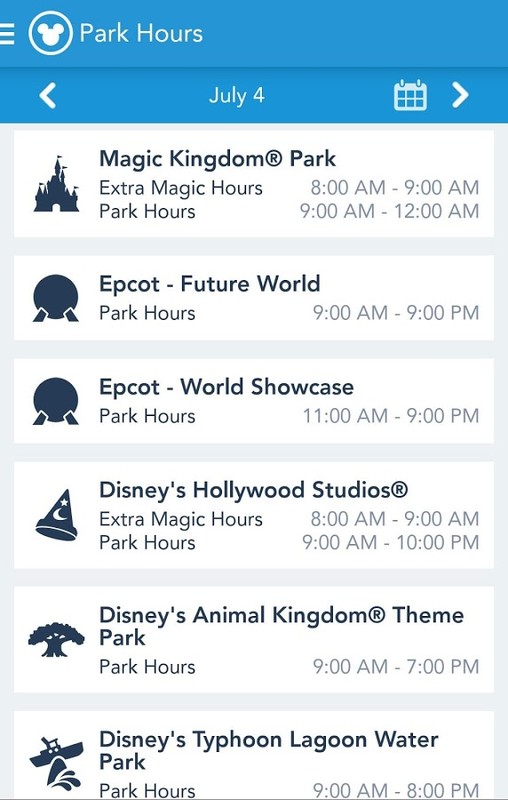A screenshot of the Disneyland app displays park hours for the 4th of July. The app shows that the Magic Kingdom Park is open from 9 a.m. to midnight, Epcot from 9 a.m. to 9 p.m., Hollywood Studios from 8 a.m. to 9 p.m., Animal Kingdom from 9 a.m. to 7 p.m., and Typhoon Lagoon Water Park from 9 a.m. to 8 p.m. The app interface features a blue header and a white background at the bottom, with grayish text. Each park listing is accompanied by an illustrative icon: a castle for the Magic Kingdom Park, a globe for Epcot, a film reel for Hollywood Studios, a tree for Animal Kingdom, and a wave for Typhoon Lagoon. The image appears to be from a mobile device, indicated by the horizontal orientation.